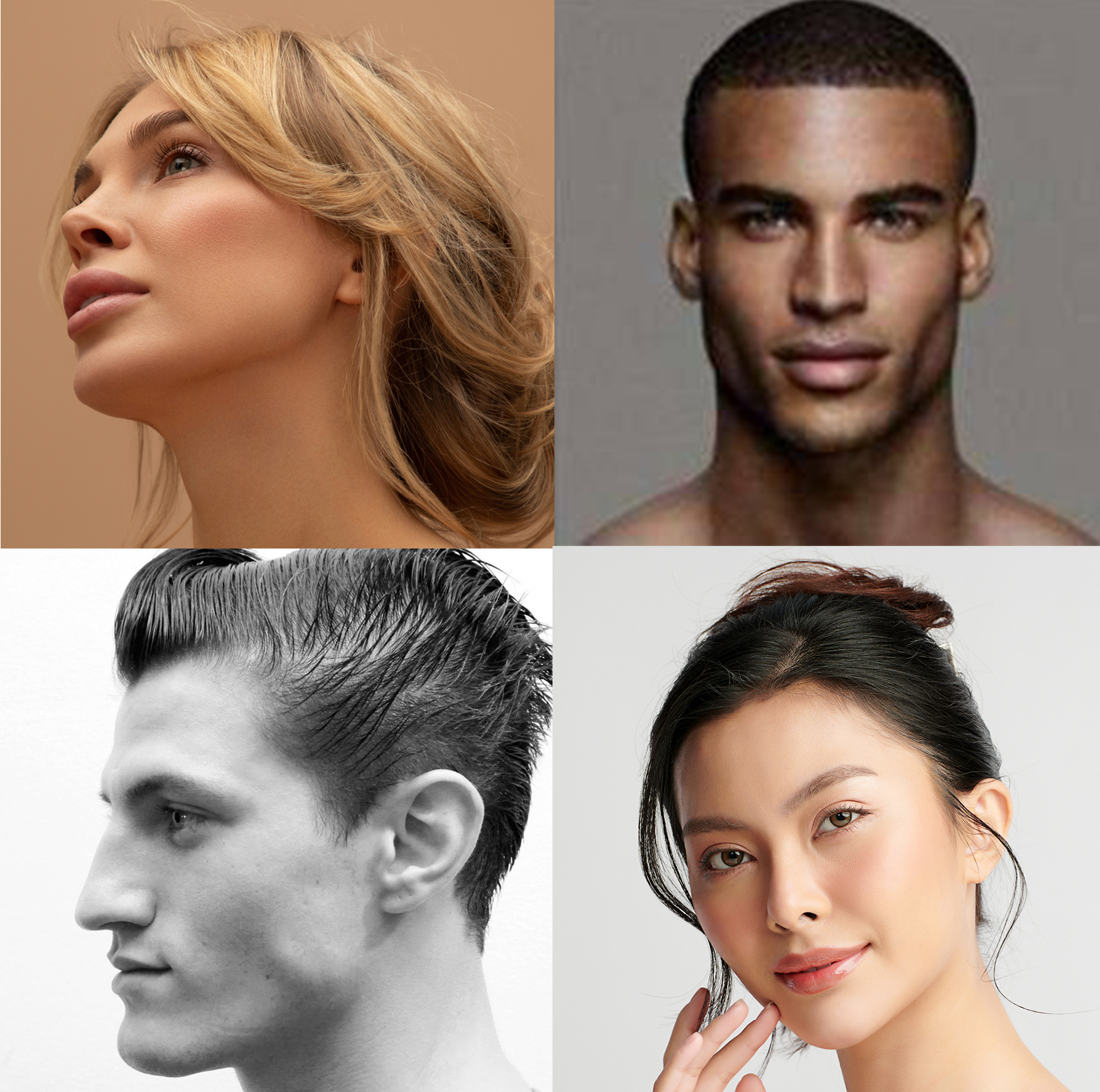The image is a collage of four headshots, each with distinct backgrounds and poses, showcasing diverse individuals. The top left quadrant features a Caucasian woman with dirty blonde hair, looking up and away from the camera against a simple beige backdrop. Her expression is neutral, and her light complexion and delicate facial features, including brown eyebrows and full lips, are accentuated. In the top right quadrant, a black man with short hair and a stoic expression faces the camera directly, set against a plain gray background, showcasing his prominent jawline. The bottom left quadrant presents a black-and-white profile headshot of a Caucasian man with dark, possibly gelled hair styled in a vintage manner. He has a lighter skin tone and high cheekbones, with a blank expression, set against a white background. The bottom right quadrant captures an Asian woman with her hair pulled into a bun, a few loose strands softening her look. She slightly tilts her head towards the camera, with a hint of a devious smile on her face highlighted by a touch of pink lipstick. Her hands are delicately positioned near her chin, with her index finger lightly touching her face, framed by a light gray background.